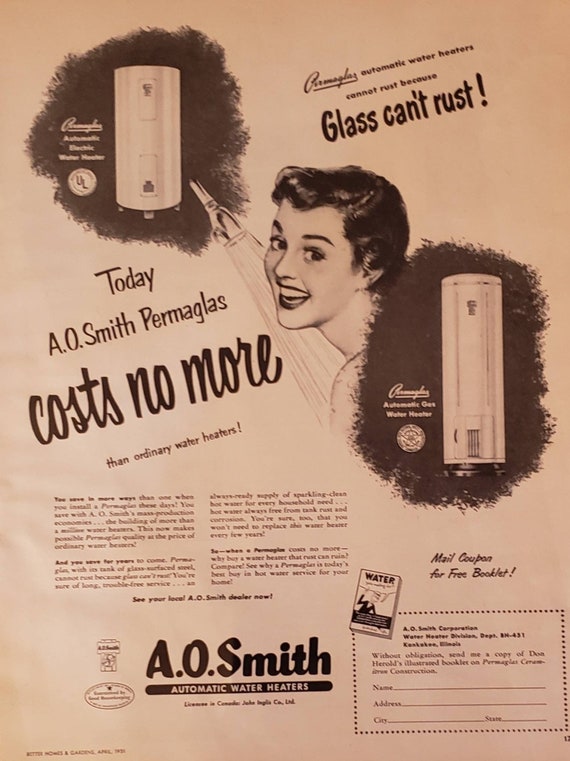This image is a black-and-white advertisement from an old, yellowed magazine page promoting A.O. Smith's Permaglass automatic water heaters. Dominating the center of the ad is a happy woman with dark hair, her head turned towards the left, smiling as shower water cascades over her. Taking up notable positions on the page are two images of water heaters, one in the top left corner and another to the right of the woman’s face, each enclosed in black shapes. 

Near the top right corner of the ad, in elegant black curly lettering, the text proudly declares, "Glass can't rust!" Below this proclamation, more text informs the reader that, "Today, A.O. Smith Permaglass costs no more than ordinary water heaters," emphasizing "costs no more" in larger letters. 

Near the bottom of the page, large bold letters read, "A.O. Smith automatic water heaters," while further down a dotted rectangle provides fields for readers to fill in their name, address, city, and state—intended for ordering a free informational booklet, the cover of which is also illustrated and labeled "Water." This booklet can be requested by mailing in the coupon, making the advertisement both an informative and interactive piece encouraging consumer engagement.